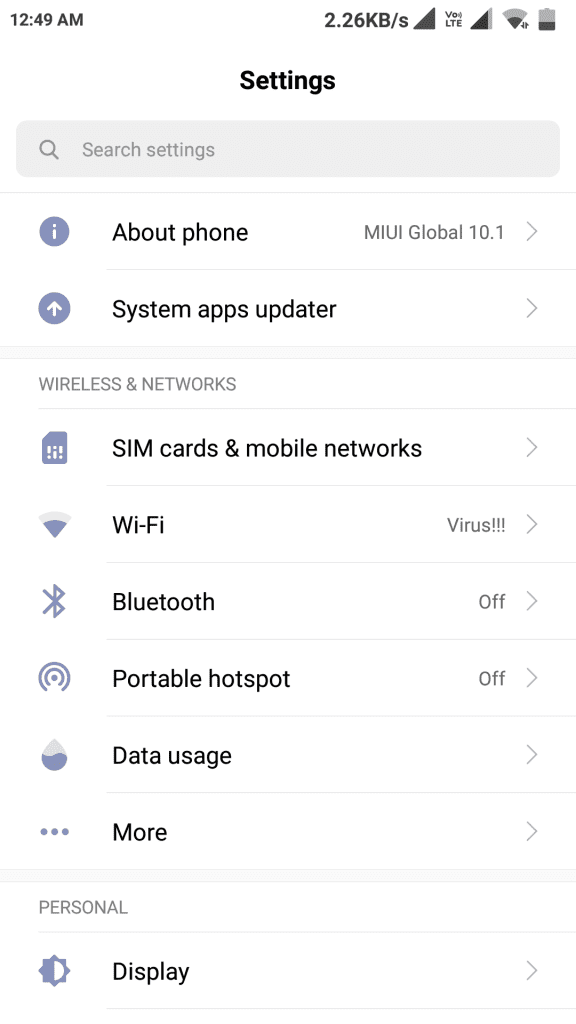The image shows a screenshot of a cell phone’s settings page taken at 12:49 AM. At the top of the screen, various status indicators are visible, including a data usage statistic of 2.26 KB/s, a triangular icon, a “VOL” indicator suggesting Voice over LTE capabilities, another triangular icon, a Wi-Fi signal icon, and a battery icon that is partially filled, indicating the battery is about a third charged and might need recharging soon.

Below the status bar is a search bar labeled "search settings." Underneath, a list of settings options is displayed, each with a gray icon on the left and descriptive text on the right. The first item features a lowercase "i" in a gray circle next to the text "About phone," followed by "MIUI global 10.1" to indicate the phone’s firmware version. The second item shows an upward-facing arrow and is labeled "System apps updater."

Further down, a heading reads "Wireless and networks," accompanied by a small card icon, followed by the options "SIM cards and mobile networks." The next visible setting is for Wi-Fi, which astonishingly is followed by the text "virus!!!," potentially indicating an issue or anomaly.

The bottom of the visible section appears to feature the "Display" setting. Each setting has an informational arrow pointing to the right, indicating further details are accessible by selecting the option.